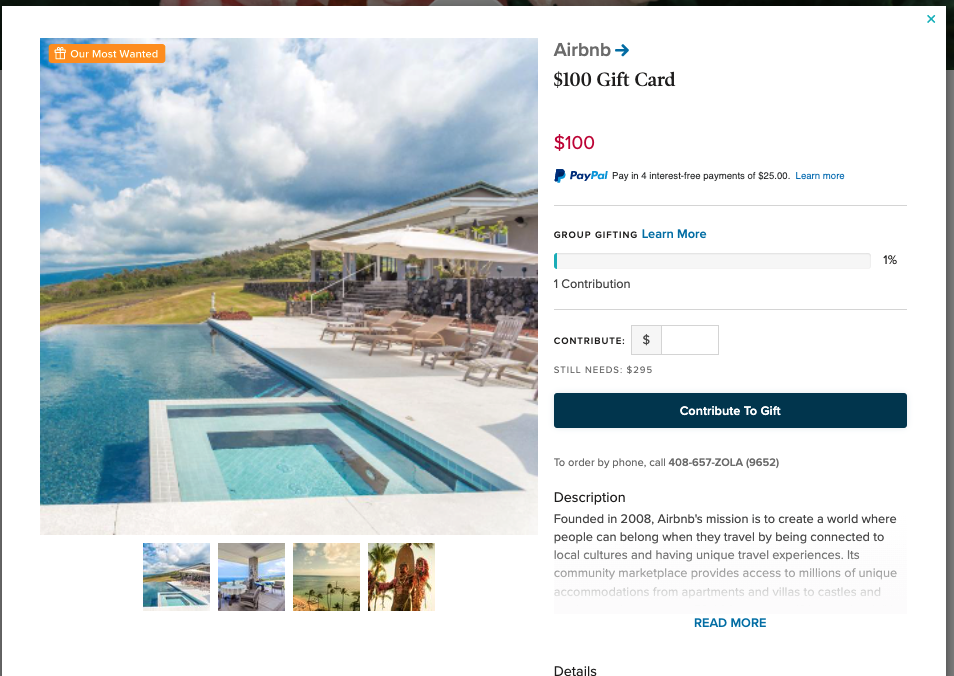This image is a detailed screenshot from the Airbnb website. The right side of the image features a section with a white background. At the very top, "Airbnb" is written in a light gray font, accompanied by a blue arrow pointing to the right. Below this, in bold black font, it says "$100 gift card," with the "$100" highlighted in red font for emphasis. Further down, the PayPal logo is displayed, with "Pay" in dark navy blue and "Pal" in sky blue, along with a stylized "P" on the left side in a navy blue and sky blue gradient. A gray text underneath describes an option to "Pay in 4 interest-free payments of $25."

Following this, the words "Group Gifting" appear, linked to a blue "Learn more" hyperlink. Below this hyperlink, there is a dark blue rectangular button with the text "Contribute to gift" in white font.

On the left side of the screenshot, there is a photograph featuring a close-up view of a serene pool area. This part of the image shows poolside lounge chairs and umbrellas under a vibrant blue sky filled with beautiful clouds. In the background, the greenery of distant trees adds a touch of tranquility to the setting.